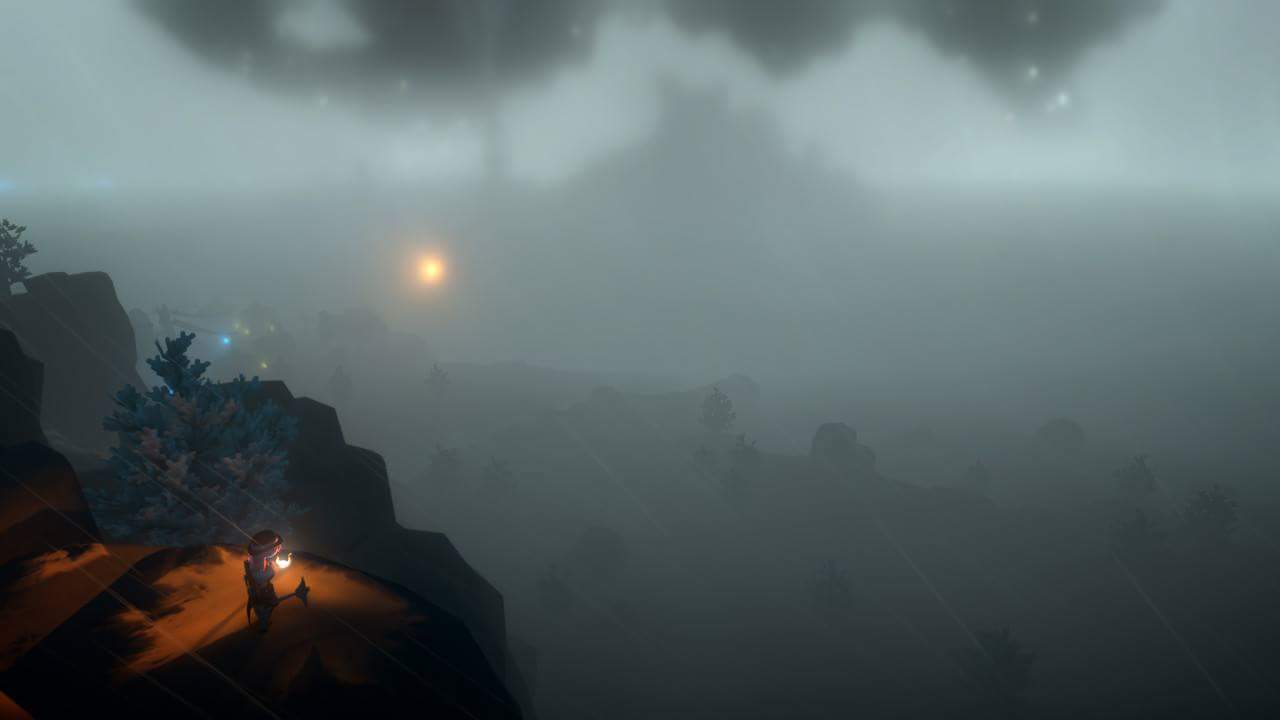This image depicts a computer-generated, video game-style scene set in a stormy, overcast, and foggy valley. In the bottom left corner, a rocky ledge adorned with coniferous trees and illuminated by a golden orange light stands out. On this ledge stands a character holding a flame torch, casting a warm glow around them. The distant landscape is shrouded in mist, with silhouettes of trees and rocks barely visible in the hazy basin below. Toward the top left, a small orange light glows in the sky. The horizon reveals a pyramid-shaped structure or mountain in the center, with a slightly lighter sky above it, and large, ambiguous dark shapes—possibly clouds or spaceships—looming overhead. On the left side of the horizon, additional light sources emitting blue and green hues add to the mysterious atmosphere of the scene.